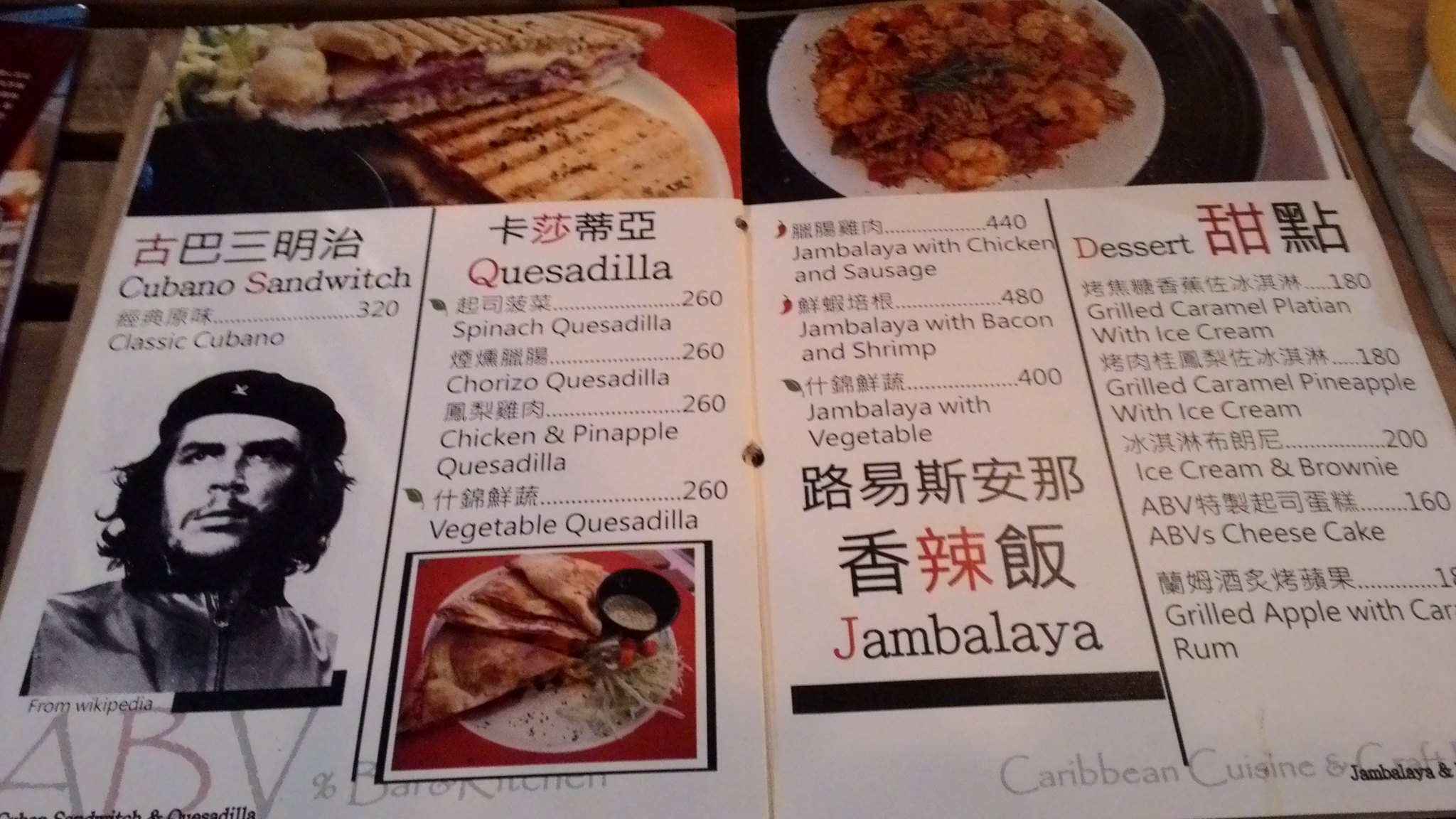The photograph features an unfolded menu consisting of two pages, each divided into two vertical sections. On the left section of the first page, there's an image of Che Guevara, accompanied by Chinese text, and the title "Cubano Sandwich." The menu item "Classic Cubano," priced at 320, is also listed here. Beneath this, there is a note indicating that the image is sourced from Wikipedia, and the initials "ABV" are displayed prominently at the bottom. 

In the next vertical section, separated by a black line, additional Chinese text is present. The item "Quesadilla" is listed with a price of 260. Sub-sections under this category include Spinach Quesadilla, Chorizo Quesadilla, Chicken and Pineapple Quesadilla, and Vegetable Quesadilla, all priced at 260. Below this, within a black square, there appears to be a photograph of a plate holding various quesadillas.

The right page's left section features "Jambalaya" with accompanying Chinese characters and prices ranging from 440 to 484. It lists varieties such as Jambalaya with Chicken and Sausage, Jambalaya with Bacon and Shrimp, and Jambalaya with Vegetables.

The final vertical section on the right is dedicated to desserts, with a comprehensive list of different dessert options, though specific items and prices are not detailed in the description provided.